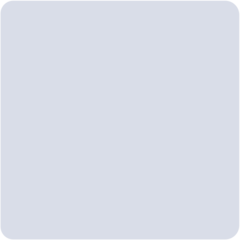A minimalist square icon with softly rounded edges, rendered in a pale, desaturated light blue hue. The color is subtly muted, giving the design a gentle and airy appearance. The overall effect is a clean and calming visual element.